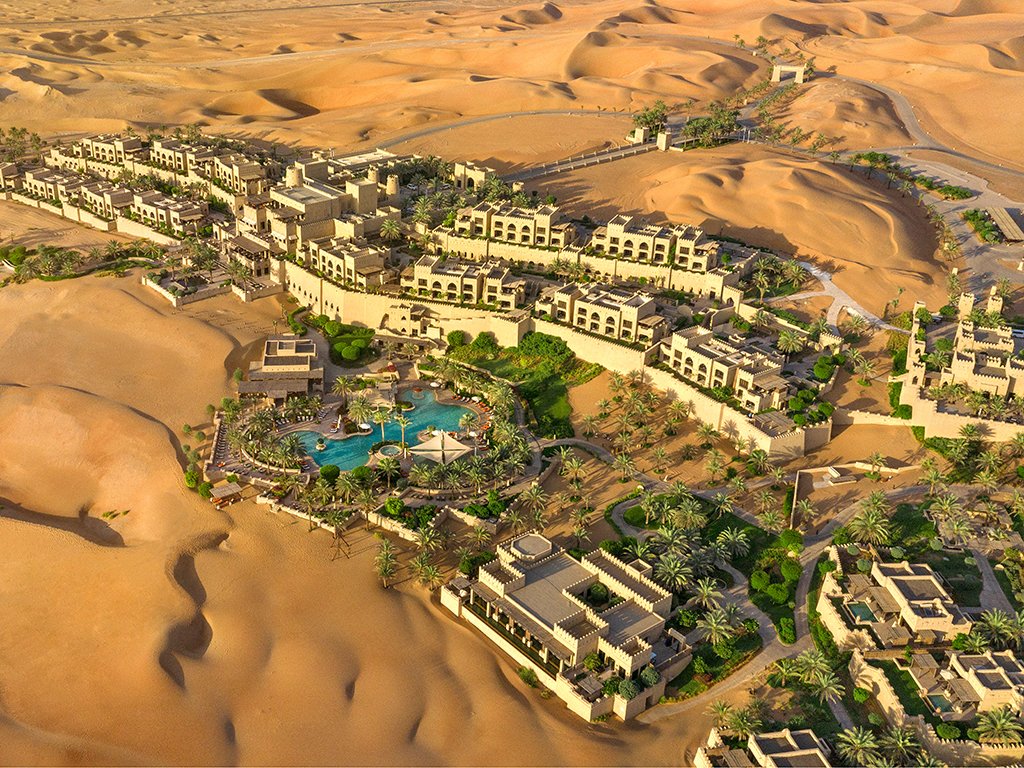The image portrays a striking oasis nestled in a vast, brown desert characterized by sweeping sand dunes. A row of elegant, white-walled buildings stretches diagonally from the upper left to the lower right of the image, resembling a village. These buildings are primarily rectangular and boxy, with some featuring distinctive castle-like tops. They appear to be part of a complex, possibly an apartment neighborhood or a hotel, given their multiple floors and numerous windows. The structures are interconnected by sidewalks and surrounded by lush green lawns, vibrant bushes, and palm trees, creating a vivid contrast against the monochromatic desert backdrop.

Central to the scene is a large, wavy pool with vibrant blue water, adding to the oasis feel. In front of the pool, to its right, and at the bottom left of the image, are additional buildings that seem to have pools of their own. The compound is enclosed by a long, white wall, and roads can be seen leading into the desert, lined with trees. Despite the presence of extensive greenery within the compound, the expanse beyond this cultivated area is entirely brown sand dunes, emphasizing the stark contrast between the cultivated oasis and the surrounding barren desert. The image is well-lit, suggesting a sunny day, though the sky itself is not visible.